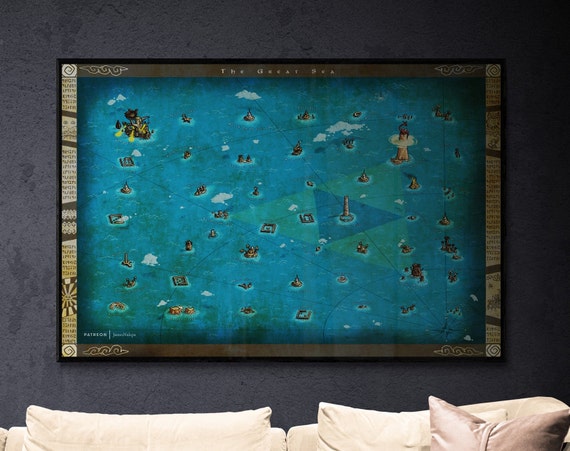The image depicts an indoor setting with a dark charcoal gray textured wall serving as the backdrop. Centered on the wall is a large, framed painting titled "The Great Sea," which is denoted in an elegant historic font at the top of the artwork. The painting features a striking oceanic scene with various landmarks like ships, towers, rocks, mountains, boats, and pillars scattered throughout. The ocean background predominantly showcases blue and green hues, with intricate visual details such as a central green and blue triangular pattern containing a circle and a pillar. The painting is framed in a combination of black and gold colors, with elaborate patterns along the sides. Beneath the painting, a light beige or cream-colored sofa is perfectly positioned, adorned with a light brown pillow on the right side of the image.